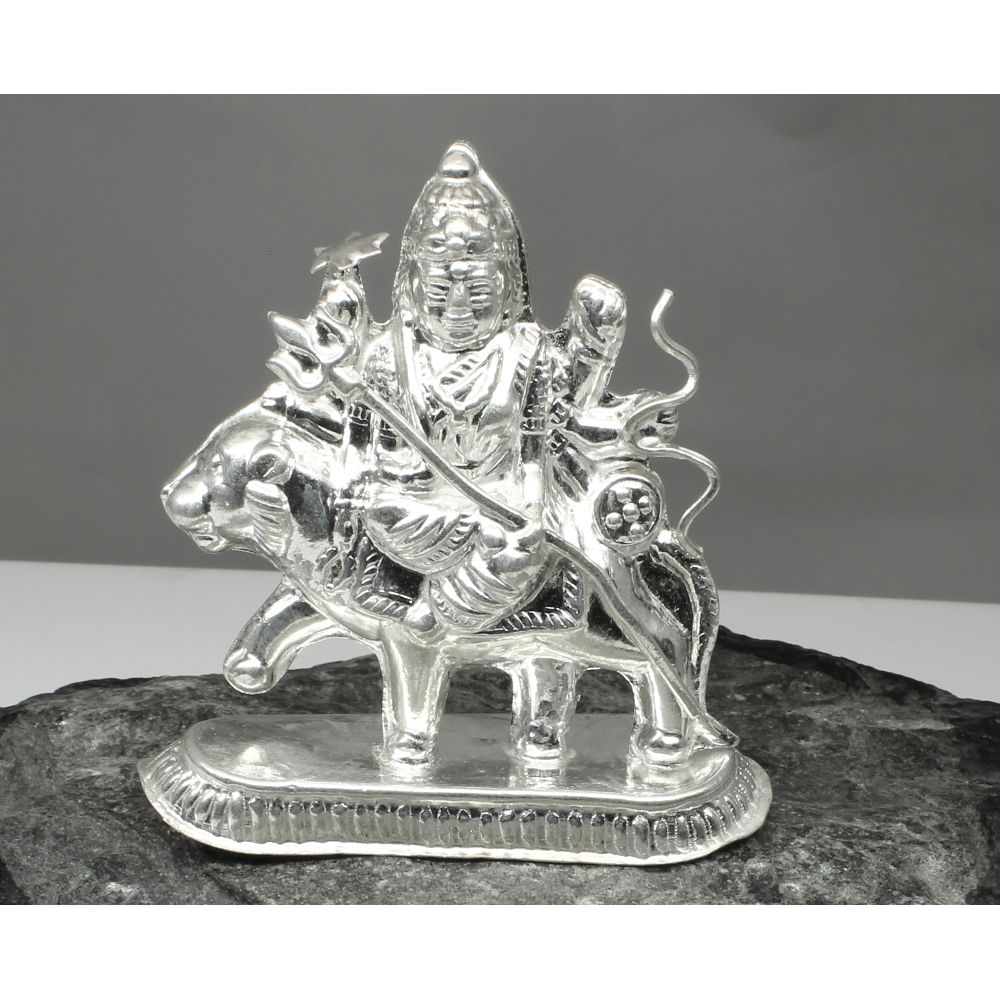The image features a detailed silver figurine, resembling an Indian deity, situated atop a meticulously crafted dark grey marble base, adorned with fine white veining. The background presents a gradient from a dark grey upper section to a lighter beige below. The deity, adorned with an ancient, conical helmet that evokes traditional masks, sits astride an animal—possibly a lion, bear, or tiger—with its right paw lifted in mid-step, creating a sense of movement. The deity holds a trident in one hand and appears to be gripping a bow in the other, facing slightly away from the majestic creature below. The base of the figurine is a flat, round plate with ridged edges, all seamlessly integrated into a single, gleaming silver composition. This intricate piece, captured in a black-and-white photograph, exudes an air of ancient mystique and craftsmanship.